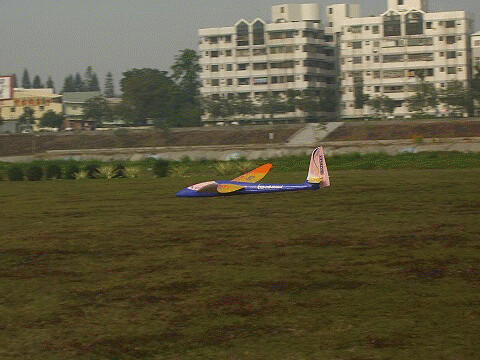The photograph captures a vibrant scene in an open, well-maintained grassy field where a remote-controlled glider is the central focus. The glider features a bright blue fuselage, orange wings with yellow and pink accents, and a white tail fin. It is positioned flat on the ground, suggesting it has either landed or is being prepared for movement. Surrounding the field at the edges are a few shrubs and a gray roadway or waterway with a ramp leading down to it. In the background, there are two tall buildings that could be apartments or condominiums, rising at least seven to eight stories high, complete with balconies and numerous windows. To the left of these structures, additional trees and a smaller building, which might be a barn or a home, are visible. The scene is devoid of people, accentuating the solitary presence of the colorful glider against the expansive, green field.